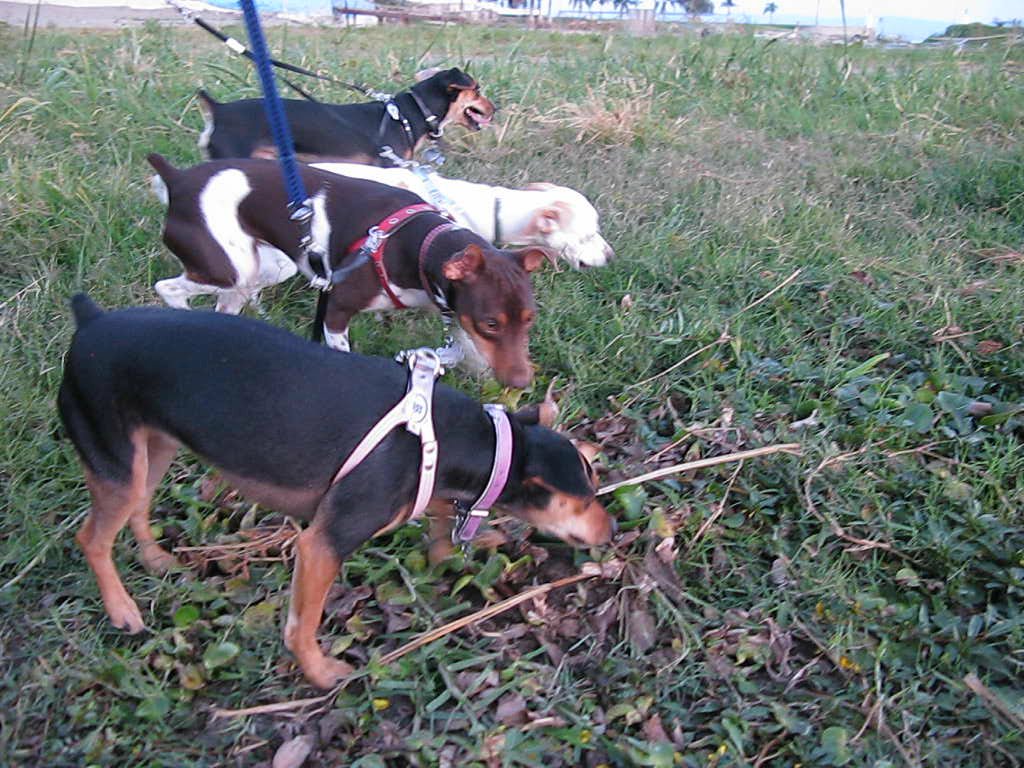In this vibrant outdoor color photograph, four medium-sized dogs of varying colors—two predominantly black with lighter orangey-brown legs, one brown with a white harness, and one white with a black collar—are seen walking through a field of grass and brush. The field is a mix of green and dried brown grasses, with hints of blue in the background suggesting the presence of a building. The dogs, who could possibly be of the same breed, are on leashes, although only three leashes are visible. The owner of the leashes is not included in the frame. The dogs appear to be proceeding forward, focusing ahead and not looking at the camera, enhancing the candid, natural atmosphere of the setting.